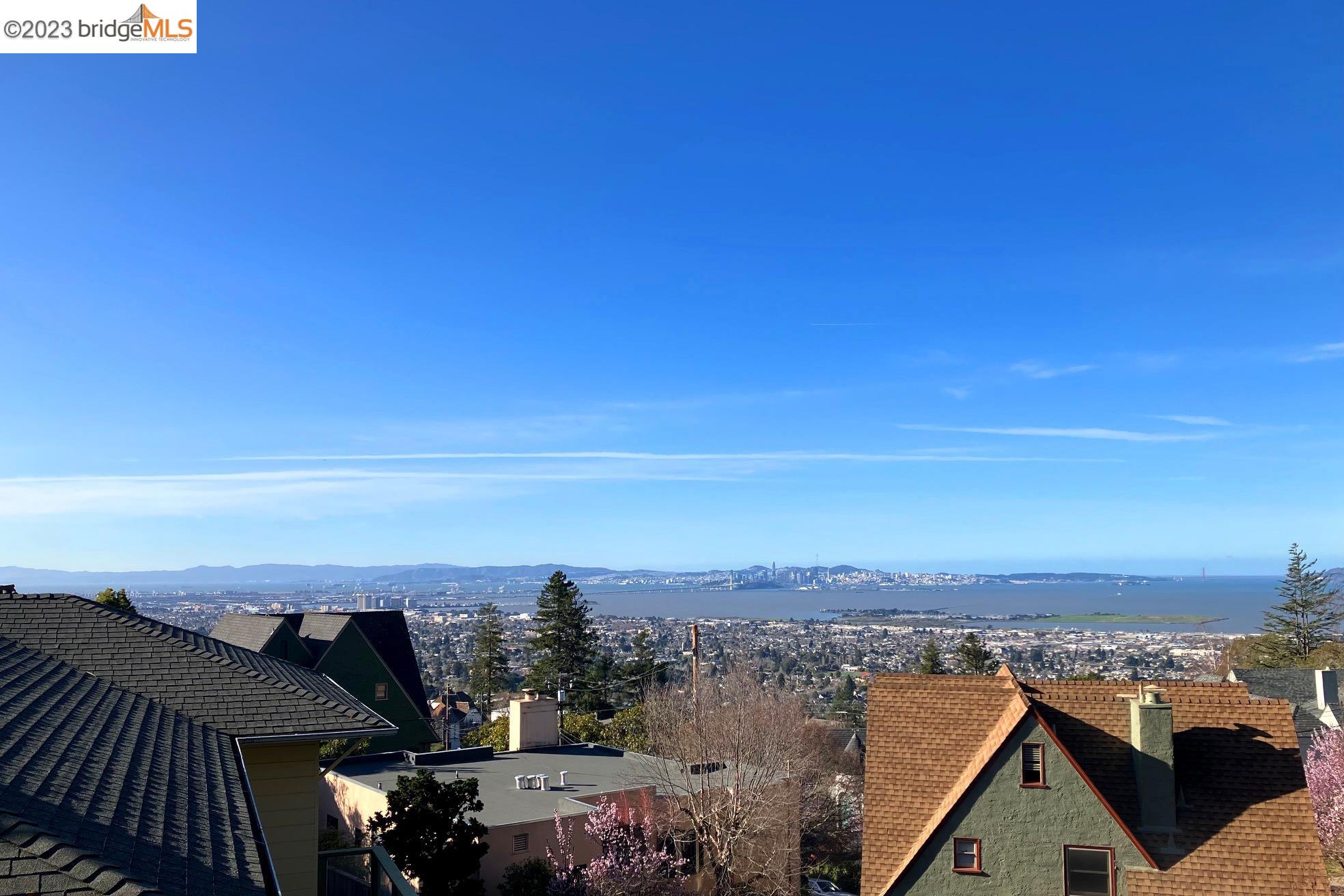This daytime photo presents a panoramic view from a high vantage point, seemingly atop a rooftop, overlooking a diverse neighborhood scene. In the foreground, rooftops of various houses are visible: a notable green three-story house with a distinctive triangular brown roof and green chimney on the right, and a partially obscured black-roofed house on the left. In the middle ground, a building with a flat roof and a nearby tree with barren branches are discernible, along with a blooming pink tree and a few scattered light poles.

Extending into the background, the view descends into a valley densely packed with trees of varying foliage. Beyond the trees, a giant lake stretches from the right towards the center of the image, bordered by lands that curve around on the left side. The farthest part of the scene features mountainous terrain and an urban landscape where multiple buildings and roads are visible. The sky above is a clear blue with wisps of white clouds scattered throughout. This photograph also bears the marking "2023 Bridge MLS" in the upper left-hand corner, indicating it may be part of a real estate listing. The composition highlights the breadth of the landscape, seamlessly integrating the immediate and distant views into a single, expansive scene.